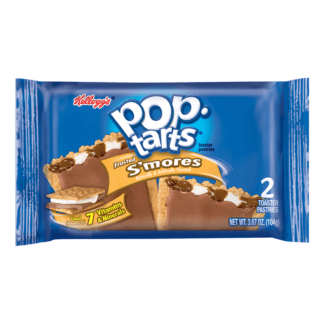A vibrant, unopened package of Kellogg's Pop-Tarts S'mores is prominently displayed. The packaging is predominantly blue, with the iconic Kellogg's logo in bold red text situated at the top left corner. The brand name "Pop-Tarts" is centered at the top in large, white lettering. Directly below, a gold banner declares the enticing flavor: Frosted S'mores. Another gold banner at the bottom left highlights the nutritional benefit, stating "7 Vitamins & Minerals" in a sleek font. In small, black text to the right of the Pop-Tarts logo, some details are barely legible. At the bottom right, in clear white text, it specifies the content of the package: "Two Toasted Pastries," and provides the net weight, "3.67 oz (104g)."